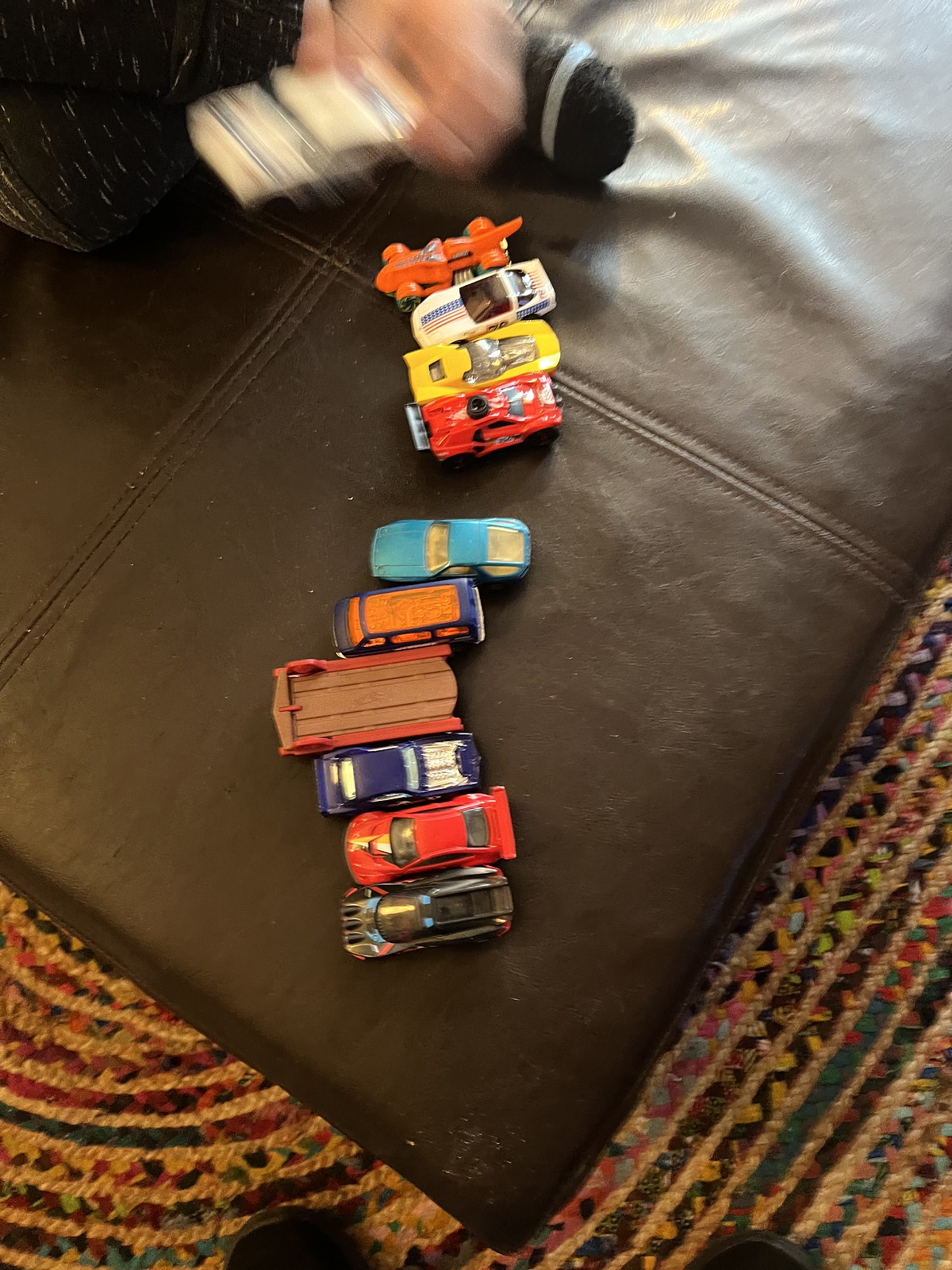The image captures an aerial view of a dark brown, chocolate-colored leather cushion situated on a multicolored, patterned rug. The rug features lines and loops in an array of colors, including green, tan, black, and yellow. Atop the cushion are nine toy cars, reminiscent of Matchbox or Hot Wheels cars, arranged in small clusters. Four of the cars are positioned close together, with a toy trailer ramp sitting centrally among them. There is a notable white toy car with blue stripes being held by a child whose presence is suggested by a partially seen leg clad in a black sock with a gray stripe. The child's hand is captured in a blur, indicating movement. At the bottom of the image, a pair of cut-off feet hint at the perspective of the person taking the picture. In the background, out of focus, appears to be another child possibly seated next to the cushion, contributing to an overall scene of playful activity.